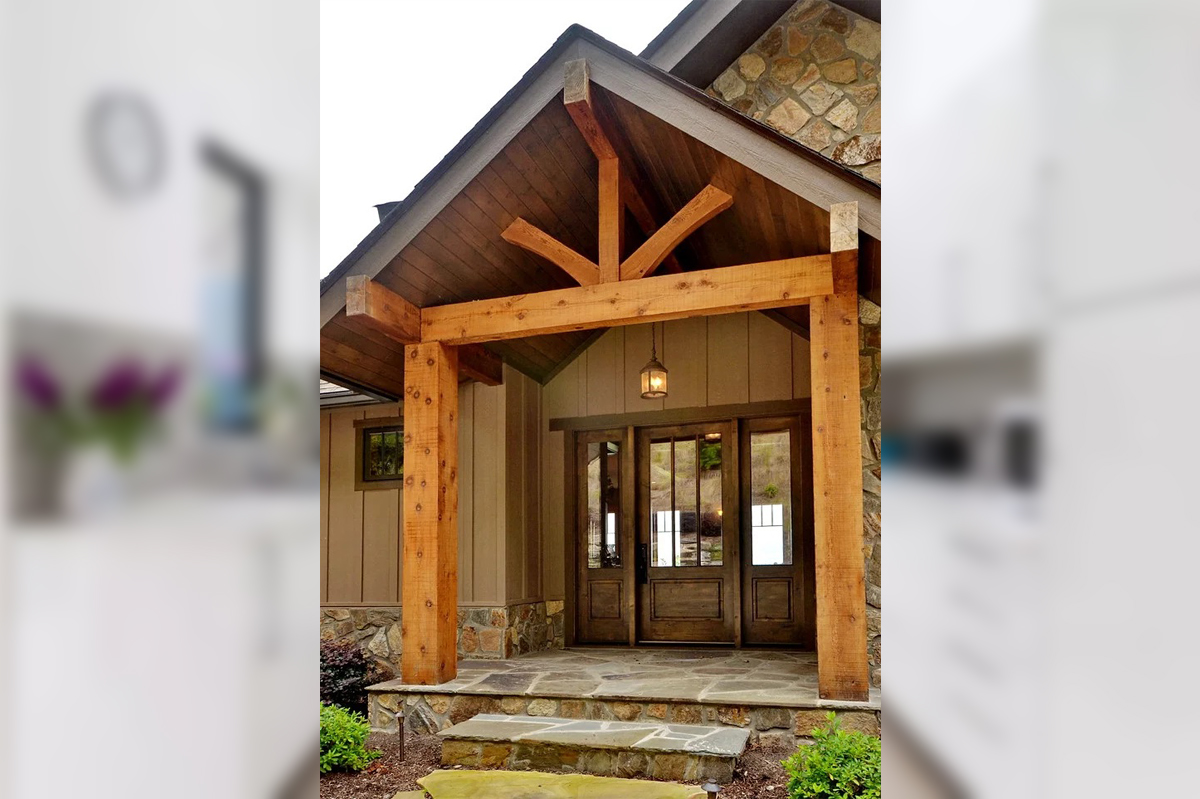The image captures the front of a beautifully rustic home, characterized by its warm, earthy tones and natural materials. The house features a quaint front porch framed by raw wooden beams supporting a small roof. A hanging porch light illuminates the entryway, casting a welcoming glow. The exterior wood siding, which runs vertically, combines shades of brown and tan, adding to the home's rustic charm. The darker stained wooden doorway boasts large vertical windows, hinting at the elegance within. This doorway is accessible via a couple of steps leading to a porch made of natural stone, contributing to its sturdy and organic feel. Surrounding the entrance, green shrubs provide touches of nature and vibrancy against the backdrop of the house's wooden and stone features. Above the porch, the higher floor showcases additional stonework, enhancing the building's cohesive and grounded aesthetic. The overall effect is a striking yet harmonious blend of natural materials, creating a cozy and inviting appearance.